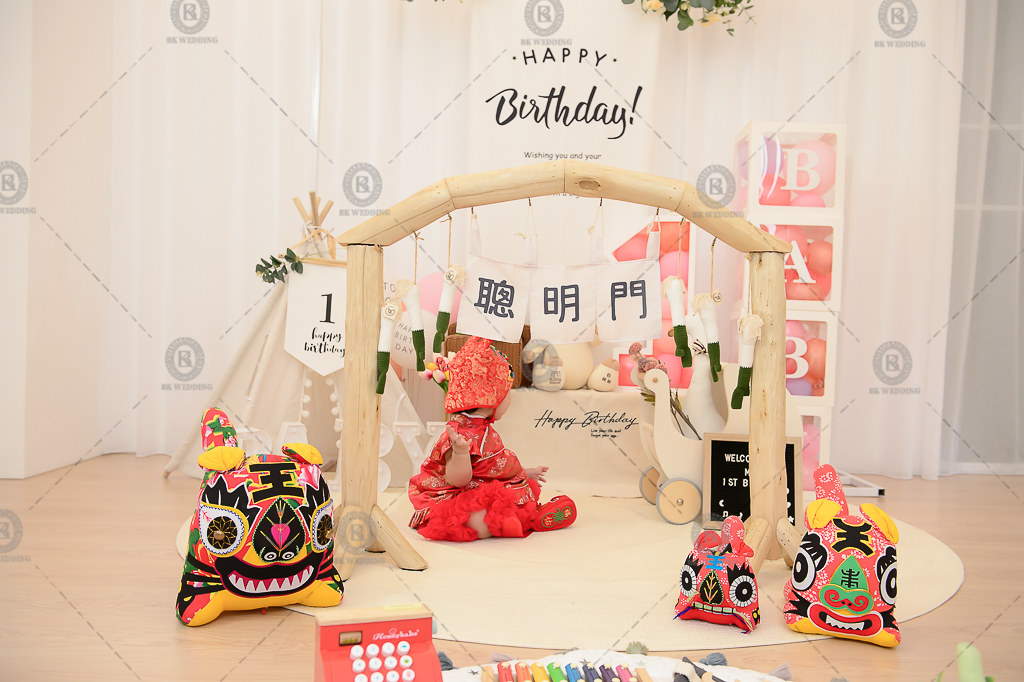This photograph captures a festive birthday setting. Central to the scene is a baby dressed in a red outfit with a matching hat, turned away from the camera, showcasing their chubby arms. They are seated on a sand-colored tile floor, surrounded by various objects. An archway structure, resembling a wooden doorway, frames the child, adorned with small flags bearing text in an unknown language. At the top of the archway, a banner reads "Happy Birthday" in bold letters. The backdrop is predominantly white with drapery and features a repeating "Happy Birthday" pattern. 

Beneath the archway lies a plush display of pillow-like stuffed animals, including a prominent red stuffed animal. Additional stuffed animals are positioned behind larger ones. Adjacent to the baby, there are decorative bags with artistic faces, including one resembling a dragon, scattered around the setup. A white wooden duck on wheels and a wooden goose on wheels are also part of the arrangement. In the foreground, the tips of colored pens can be seen, suggesting a creative element. A small shelf with various tchotchkes and toys sits behind the baby, further enhancing the celebratory atmosphere. Off to the middle right, the edge of a flower bouquet with yellow blooms adds a subtle touch of color and nature to the overall scene.